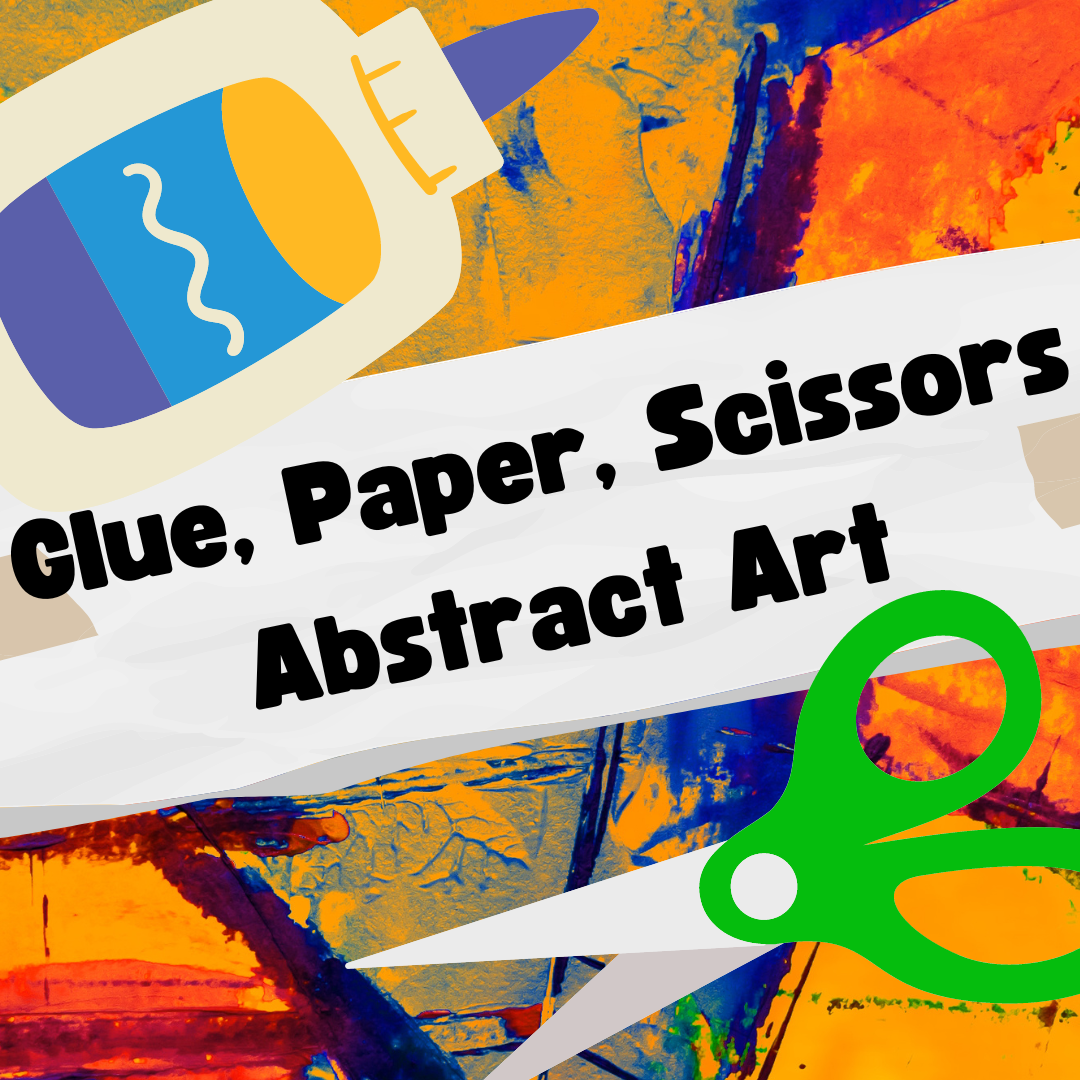The image is a stylized color illustration, resembling a kindergarten classroom poster, depicting a simple representation of a glue bottle and a pair of scissors. The glue bottle, located in the top left, is off-white with beachy colors like gold, blue, and purple, featuring a label resembling a barrel with dark blue, light blue, and yellow bands, and a white squiggle in the middle. The scissors, situated in the bottom right, have gray or white blades with bright green handles. Across the center, a banner reads, "Glue, Paper, Scissors, Abstract Art," on a slight diagonal from left to right, set against a white background with black text. The overall backdrop of the image is a vivid and angular abstract design with thick, impasto-like paint textures in various hues of orange, yellow, blue, and red, adding to the poster's dynamic and artistic feel.